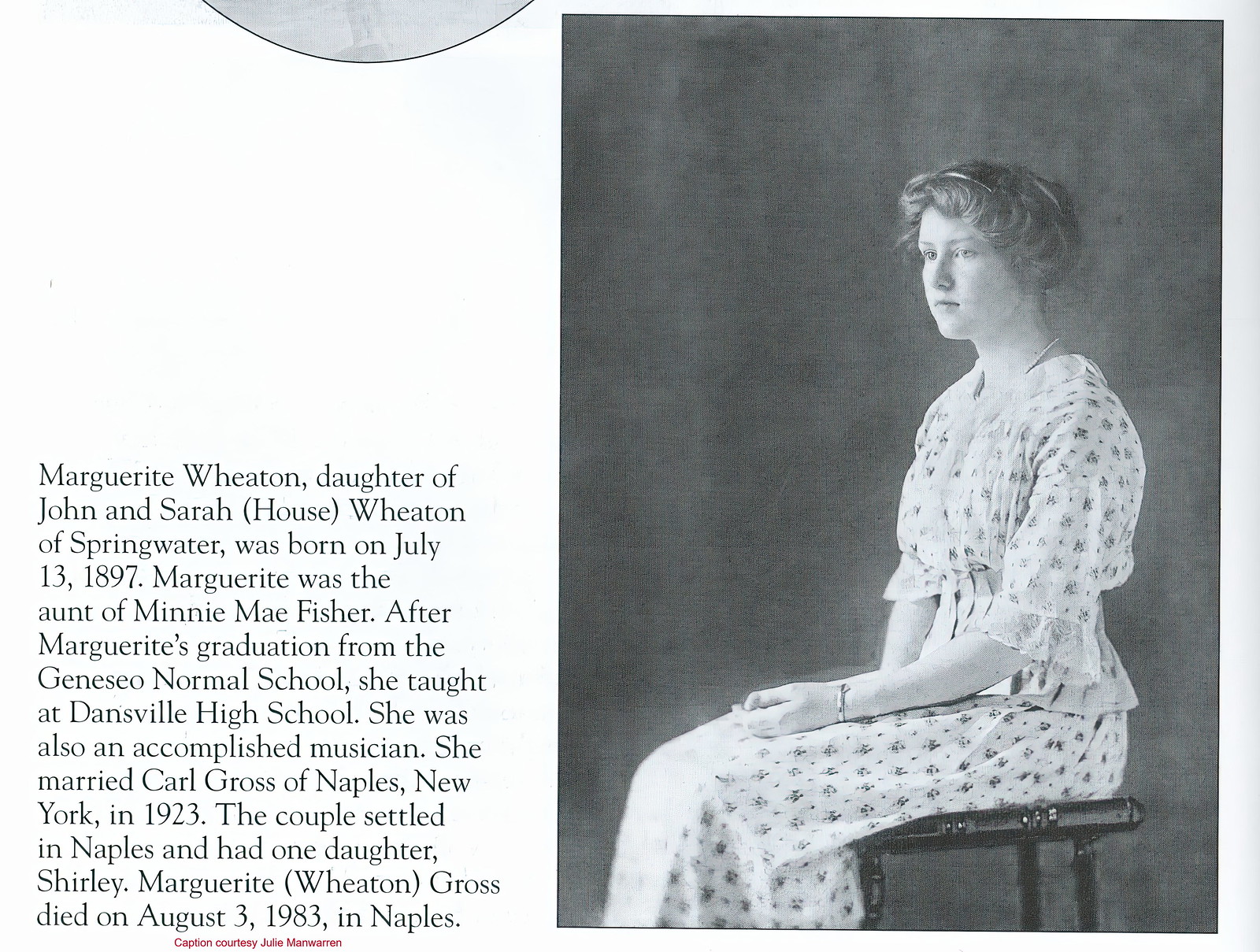This faded, black-and-white image seems to be a page from a magazine or a textbook, possibly serving as a memorial. On the right, a young woman, Marguerite Wheaton, is seated in a side profile on an ornate, thin-legged black wooden chair. She wears a light-colored dress adorned with a delicate floral pattern and lace on the sleeves. Her hair is upswept, featuring a small hairband, and she has an emotionless expression as she gazes into the distance with her hands resting in her lap. The background is gray, enhancing the contrast between her light dress and the dark chair.

To the left of the image, there is black text on a white background providing a detailed biography. It reads: "Marguerite Wheaton, the daughter of John and Sarah House Wheaton of Springwater, was born on July 13, 1897. Marguerite was the aunt of Minnie Mae Fisher. After her graduation from the Geneseo Normal School, she taught at Danville High School. She was also an accomplished musician. In 1923, she married Carl Gross of Naples, New York. The couple settled in Naples and had one daughter, Shirley. Marguerite Wheaton Gross died on August 3, 1983, in Naples." The graininess of the photograph and the reverent tone of the text suggest the image is quite old, adding a timeless quality to this homage of Marguerite's life.